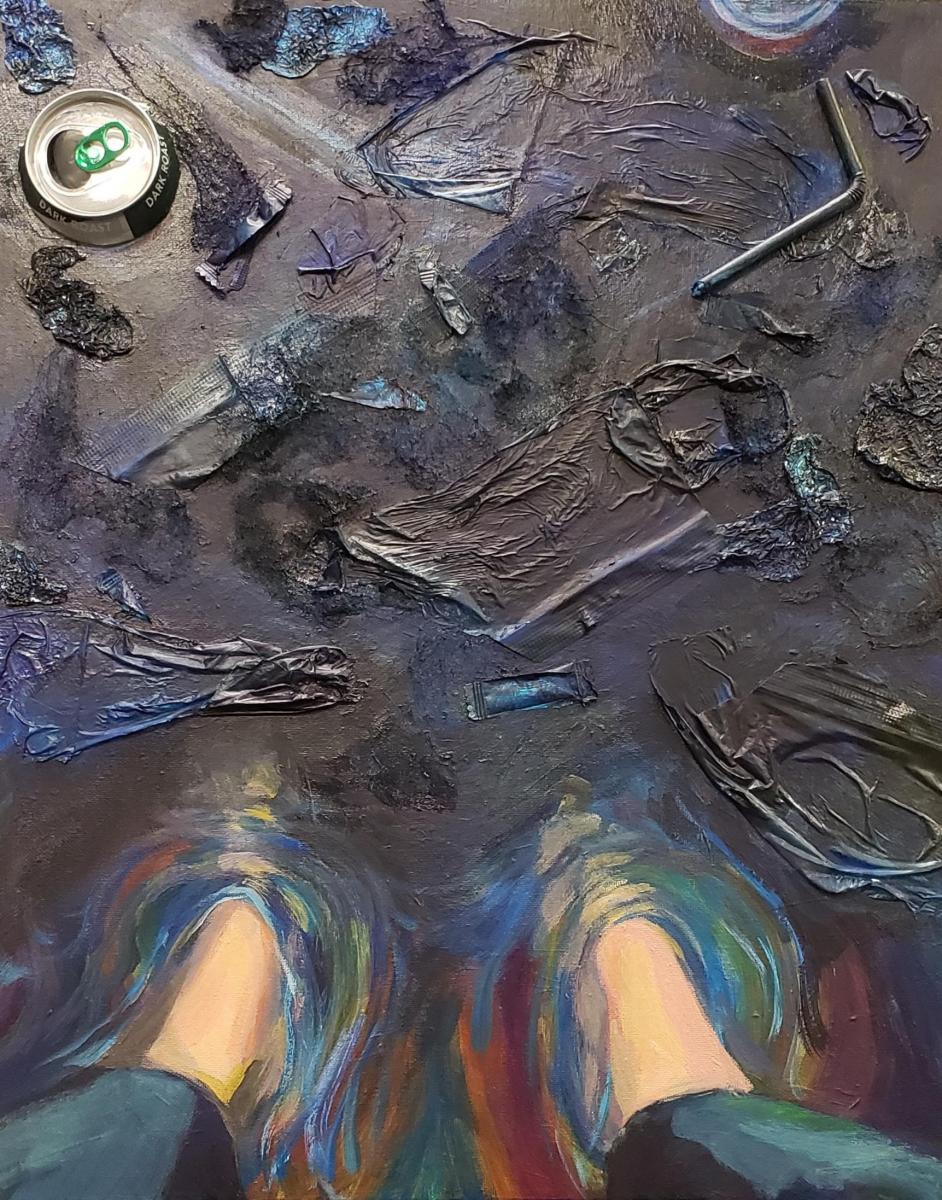This mixed-media oil painting depicts a poignant scene viewed from the perspective of an individual looking down at their bare feet, situated in a shallow pool of murky, ankle-deep water strewn with an assortment of trash. The person, clothed in dark blue trousers rolled up to reveal their skin, stands immersed in a contaminated mix of mud and garbage. The diverse debris floating around their feet includes old aluminum cans, plastic straws, wrappers, pieces of metal, tissue, a Ziploc bag, a ketchup packet, and a grocery bag. The liquid surrounding the feet exhibits a swirl of muted colors—bluish, purple, green, red, and orange—against a backdrop dominated by dark, ugly browns and blacks, enhancing the painting's dismal atmosphere. Notably, an aluminum can is embedded into the top left corner of the artwork, further emphasizing the mixed-media approach and the overarching theme of pollution and neglect.